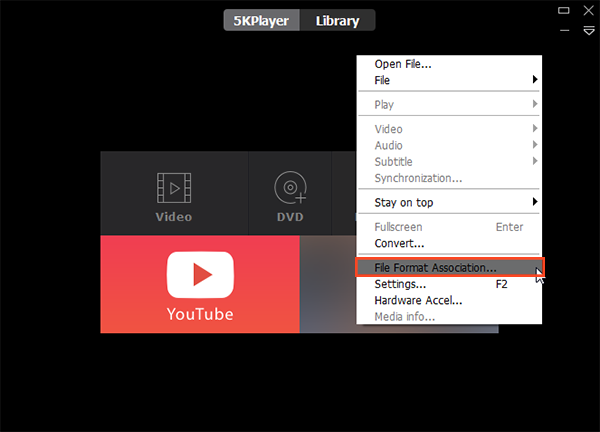This screenshot displays a desktop application designed for downloading and storing YouTube videos. The interface features a predominantly black background, with "5KPlayer" clearly labeled at the top of the library section. Beneath this, the main navigation bar includes options such as 'Video' and 'DVD,' along with a prominent red button labeled 'YouTube.'

The right-click context menu is open, presenting various functionalities like 'Open File,' 'Play,' 'Video,' 'Audio,' 'Subtitles,' 'Synchronization,' 'Stay on Top,' 'Full Screen,' 'Convert,' 'File Format Association,' 'Settings,' 'Hardware Acceleration,' and 'Media Info.' The mouse pointer is currently clicked on the 'File Format Association' option, which is highlighted in a red box.

This setup suggests that the program is demonstrating how to download and change the file format of YouTube videos. The clear distinction of color, with the mostly black interface contrasted by the red YouTube icon and red-highlighted options, simplifies navigation. This desktop application is aimed at users looking to manage digital media on their computers.